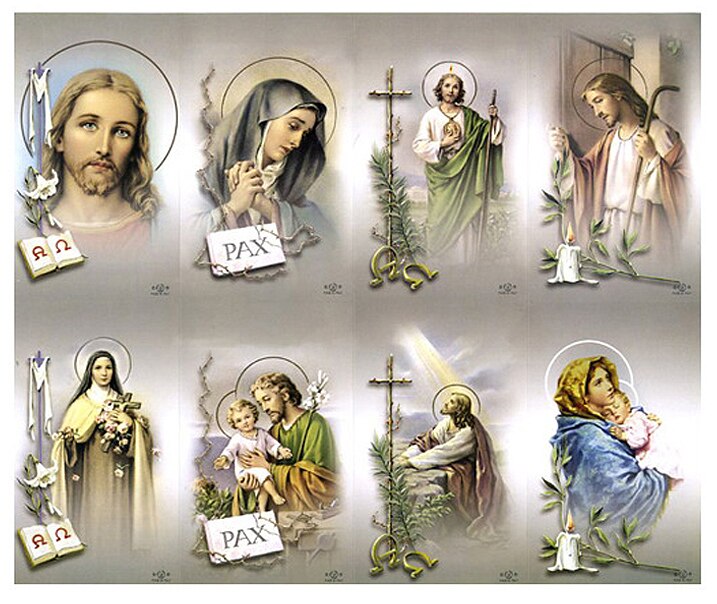The image is a collage-like poster featuring eight distinct religious depictions, organized in two rows of four against a gray background, each adorned with a halo above the figures' heads. The characters are vividly colored, enhancing their prominent features. 

In the top left corner, there is an image of Jesus Christ looking upwards with a book open in front of him, displaying two Greek letters, possibly representing Alpha and Omega, and a small white flower. Next, to the right, is a sorrowful-looking female figure, likely the Virgin Mary, holding a white board with the word "PAX" inscribed at the bottom. The third image in the top row portrays Jesus standing, dressed in a white robe and green sash, with a large cross nearby and holding a staff embellished with Greek letters. In the top right, another image of Jesus shows him holding a plant and a staff, accompanied by a candle.

The bottom row starts with a possible depiction of Mary, clothed in a yellow robe and headscarf, holding a cross among flower petals, with a book displaying Greek letters beside her. Following is a bearded man, possibly Jesus, with shorter hair, cradling a baby in a pink shirt, with the word "PAX" inscribed below. Third in this row is Jesus kneeling near a rock, gazing up towards the sky with rays of light illuminating him, beside a cross and palm trees. Finally, the bottom right features a woman, possibly Mary, with a yellowish-brown shawl, holding a baby in a light pink shirt, with a lit candle and plant below, also accompanied by Greek letters.